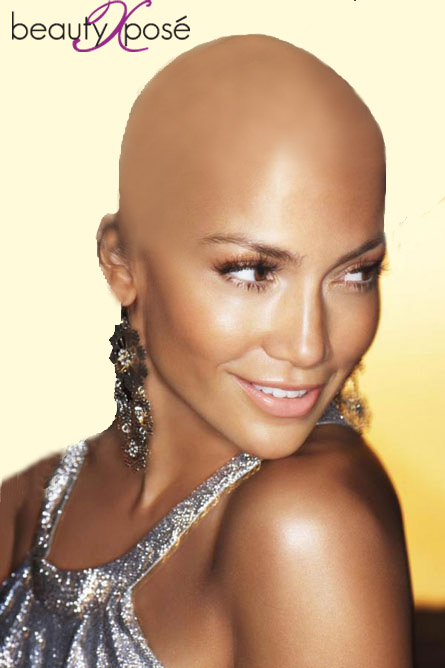This professional close-up photograph captures a bald, dark-skinned woman with a radiant, brown complexion. She is slightly smiling, revealing her front teeth, and looking to the right while tilting her head over her shoulder. She has a fully shaved head and is adorned with long, dangly earrings that reach down to her neck. Her makeup is meticulously applied, with prominent mascara and long eyelashes. She's wearing a glittering, silver-colored halter neck top that sparkles brilliantly in several places. The background is a gradient of cream and yellow, with the phrase "Beauty, Pose, Beauty, Pose" written in the top left corner.